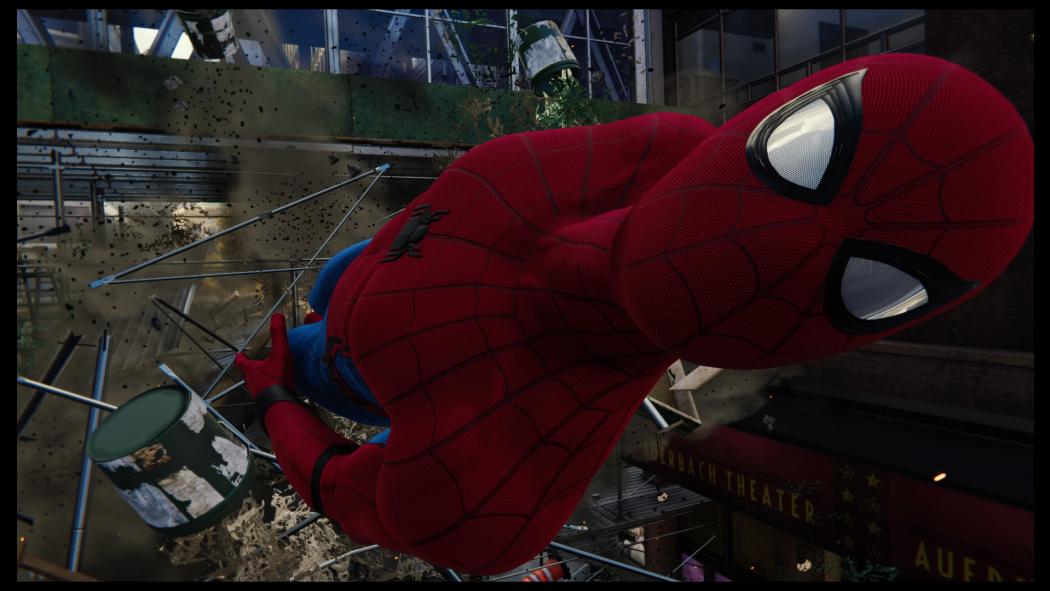The image is a highly detailed rendering from the Spider-Man video game, showcasing impeccable graphics. Spider-Man, donning his iconic red and blue suit with black webbing and white eyes, is prominently featured in the frame. His head is positioned in the upper right corner, moving towards the center, and his body appears parallel to the bottom of the frame as if he is flying or swinging toward the viewer. His suit, with its distinct red top and blue pants, also includes the familiar spider emblem on his chest. 

In the background, there is a chaotic scene with metallic scaffolding and various structures—likely a gritty warehouse—featuring numerous middle pillars, containers, and dirt scattered around. Notably, a green paint can is visible near his left hand, with paint spilling out, suggesting dynamic action as he navigates through the scene. Above this can, there are cylindrical objects and poles, adding to the industrial setting. Additionally, the bottom right of the image displays text that hints at a theater, indicating the environment is urban and possibly under construction or renovation.